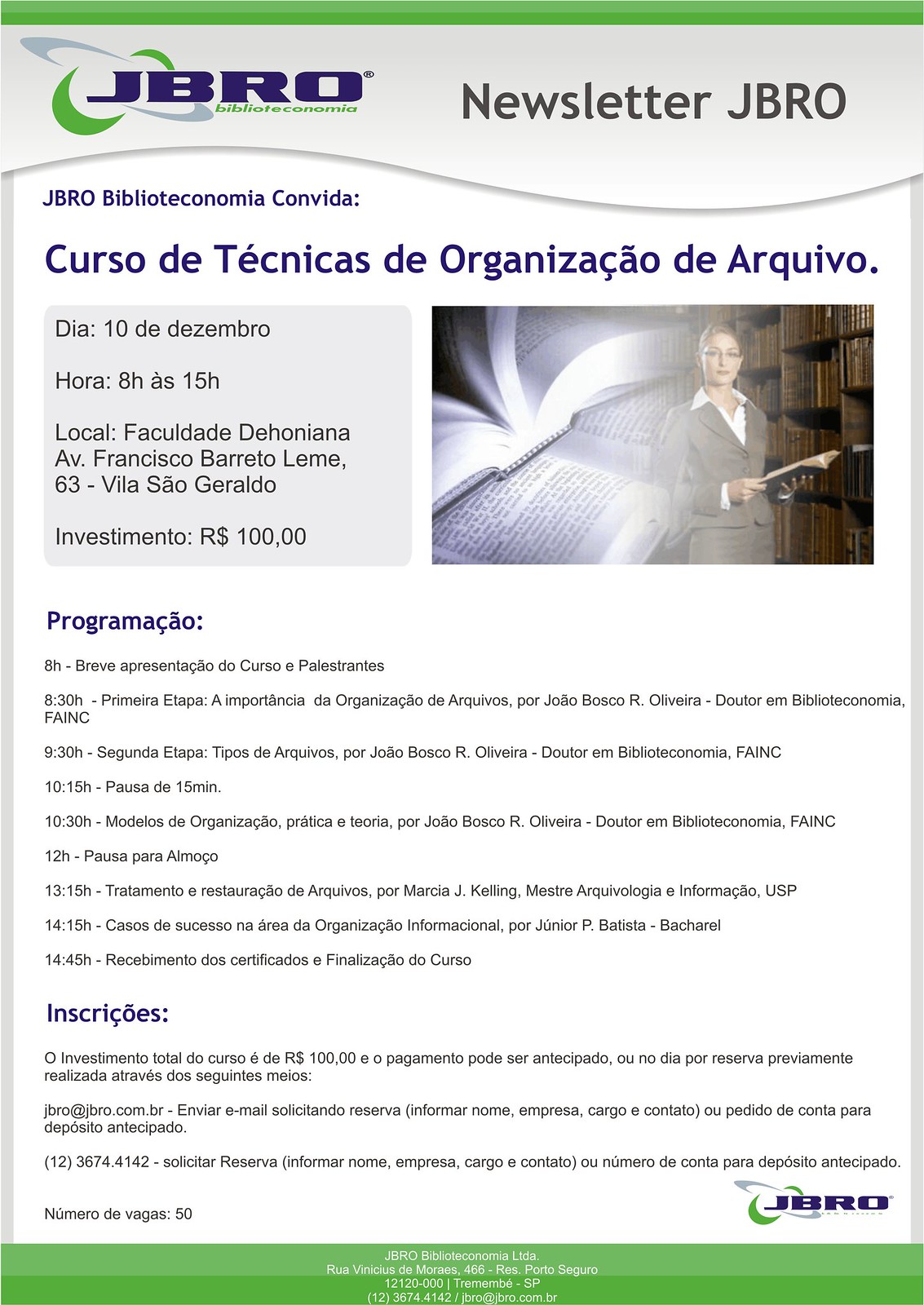The front cover of the JBRO newsletter, titled "Newsletter JBRO," is richly designed with green stripes on the top and bottom. Displayed prominently at the top is the JBRO logo in blue, alongside the phrases "JBRO Biblico Tincon Con Vida" and "Biblioteconomia," indicating a focus on library science. The language of the newsletter and program details is Spanish, featuring a comprehensive list of program times and information under headings like "Dia," "Hora," "Local," and "Investimento." Centrally, there is a striking image of a woman standing in a library. She is wearing a brown skirt and jacket paired with a white collared shirt, her hair pulled back in a ponytail, and glasses enhancing her professional look. The woman holds an open book, symbolizing knowledge and learning, with the overlaid imagery of two open books beside her, further emphasizing the theme. Additional contact information, including an email (JBRO@JBRO.com.br) and a phone number [(12) 3674-4142], as well as a location address (JBRO 466 Porto Sergo 12120-000), is provided at the bottom of the cover.